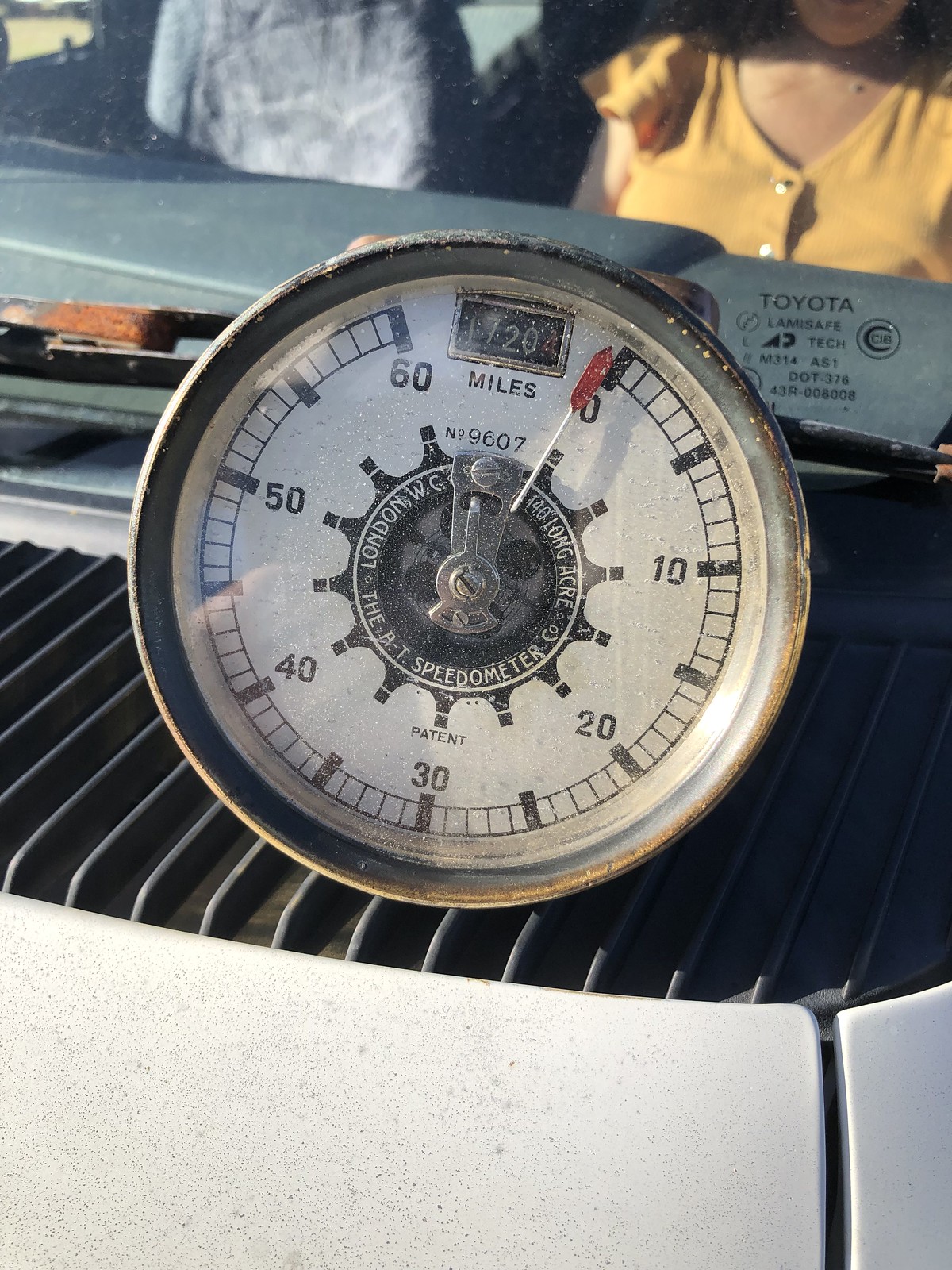The image captures a vintage speedometer with a prominent white face and a silver hand tipped in red, which spans a speed range of 0 to 60 miles per hour. Centrally located within the speedometer, there is an odometer displaying "20 miles," with the word "miles" clearly labeled underneath. Surrounding the center of the dial are various text, including "London, WC" and "AT Speedometer." Additionally, there is a small logo on the middle right of the dial bearing the name "Toyota" and some indistinguishable text following it. The speedometer appears to be mounted on a grate-like surface, reminiscent of a car's interior. In the background and partially visible through the edges of the instrument cluster, there are two individuals: a woman wearing a yellow shirt and another person dressed in a gray shirt, adding context to the photo's setting.